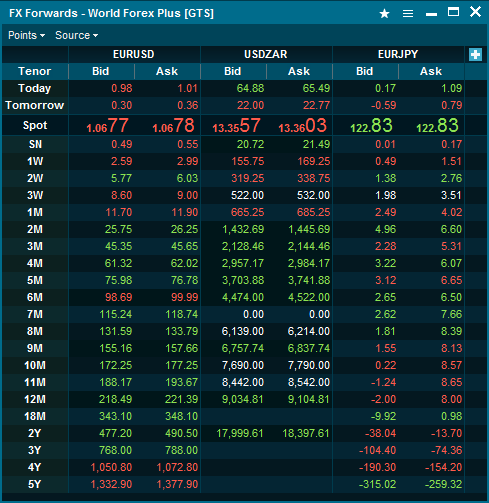The image is a screenshot of a trading platform's interface, although it is not clear whether the platform is being viewed on a tablet or a phone. At the top of the screen, there is a blue bar with white text that reads "FX - Forwards World 4x Forex Plus (GT)". To the right of this bar, there are several icons: a star, three horizontal lines, a single line, a square, and an X.

Below this top bar, there is another bar with drop-down menus labeled "Points" and "Source." Following this, there are three categories displayed: "EUR/USD," "USD/ZAR," and "EUR/JPY." To the right of these categories, there is a blue box with a white plus sign inside it.

Underneath these categories, there is another bar titled "Tenor." For each currency pair (EUR/USD, USD/ZAR, EUR/JPY), bid and ask prices are listed in two lines: one labeled "Today" and the other labeled "Tomorrow." For example, the bid price for EUR/USD today is displayed as 0.98 in red, while the ask price is 1.01. For tomorrow, the bid price for EUR/USD is 0.30 in red, and the ask price is 0.36 in red.

The list continues under the titles "Today" and "Tomorrow," extending to additional intervals such as "Spot," "SN," "1W" (one week), up to "5Y" (five years). For instance, under the 4M (four months) category for EUR/USD, the bid price is 61.32 in green, and the ask price is 62.02 in green. These details are repeated for all listed currency pairs across the different time intervals.